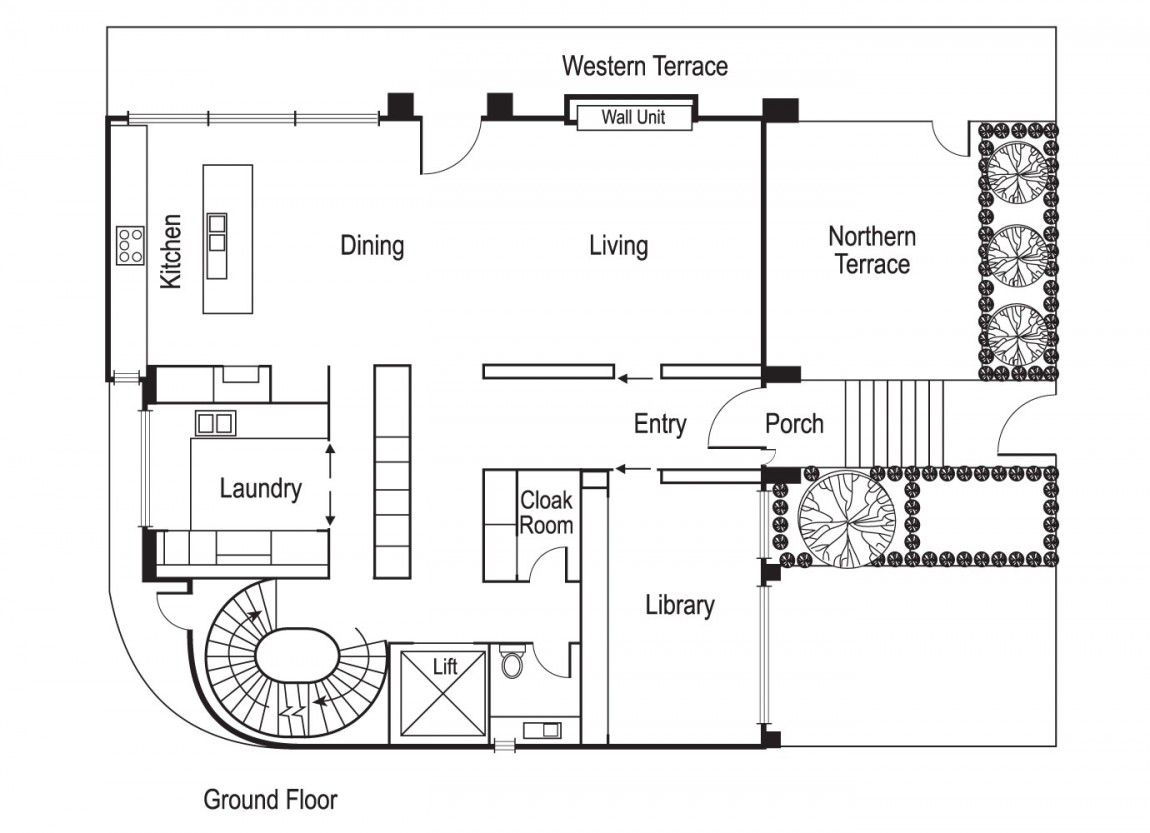This detailed architectural drawing depicts a rectangular home with a distinctive layout, rendered in black and white. The illustration is wider than it is tall, with a unique curved corner on the lower right, contrasting with the otherwise straight lines of the structure. 

At the top of the drawing, "Western Terrace" is prominently labeled, delineating an outdoor section aligned with the house's border. The layout showcases an open-plan design in the upper left quadrant, where the kitchen seamlessly transitions into the dining room and living room. An accessible door is positioned above this open space, leading outside.

On the right side of the upper section, labeled "North Terrace," the design includes space allocated for three plants against the border, adding a touch of greenery to the schematic.

The lower section of the drawing highlights various functional areas. Starting from the left, there is a laundry room adjacent to a spiral staircase. Below the staircase lies a segmented area, featuring a cook room and a lift, likely an elevator. A central hallway bisects this lower section, with stairs noted within this corridor, leading out to a porch.

In the middle lower part of the drawing, a library is situated, contributing to the home’s intellectual and leisure spaces. Another outdoor area appears in this section, complete with a plant and additional elements for outdoor activities. The intricate layout and thoughtful design details present a comprehensive overview of this sophisticated home.